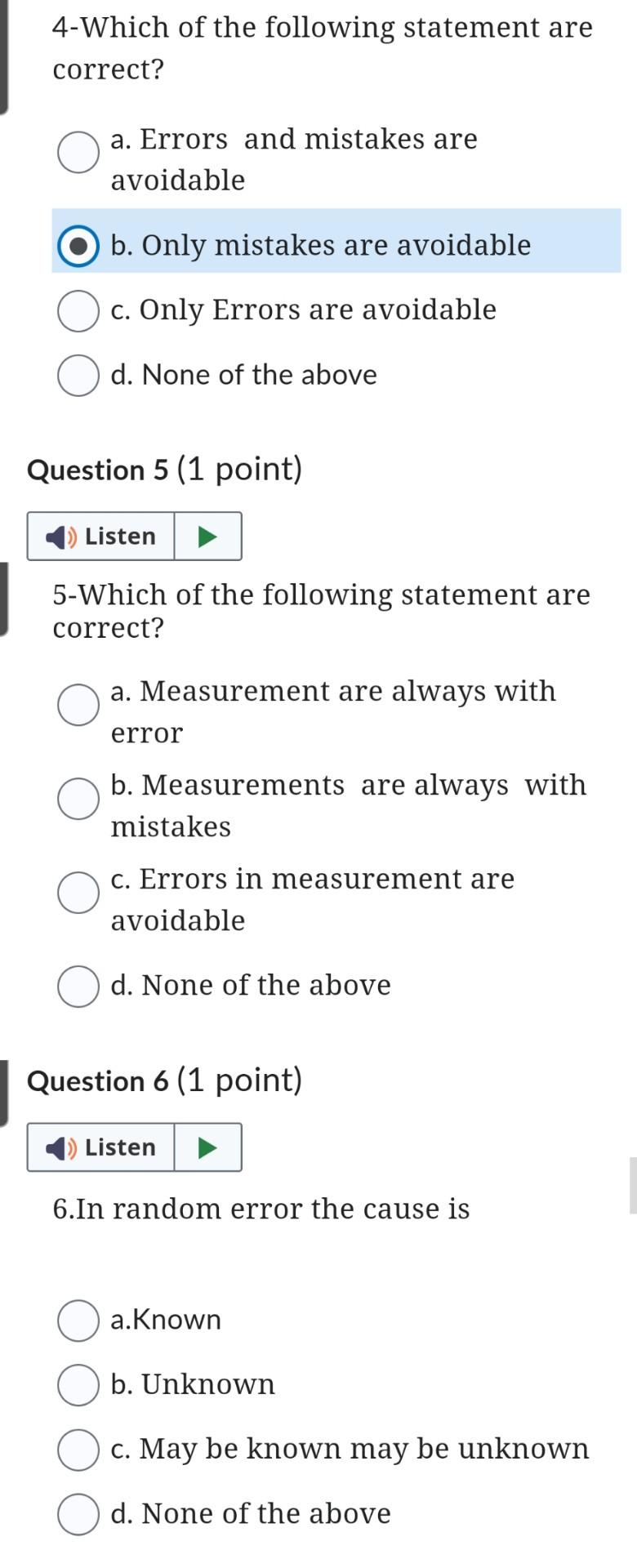The image is a screenshot taken from a mobile device with dimensions typical of a cell phone, characterized by its much taller-than-wide aspect ratio. The background of the screenshot is predominantly white, and it features black or dark grey text for readability.

The screenshot displays a portion of a quiz or survey with three visible questions, each accompanied by four possible multiple-choice answers in the form of bubbles labeled A, B, C, and D. To select an answer, a user must tap one of these bubbles next to the appropriate letter.

Additionally, beneath each question is a "Listen" button with a speaker icon, followed by a green play button with a right-pointing arrow, enabling audio playback of the question which assists in answering.

The details of the questions are as follows:
1. **Question 4**: The text reads, "Which of the following statements are correct?" The user has selected option B, labeled "Only mistakes are avoidable."
2. **Question 5**: This question prompt indicates that it is necessary to listen to the audio to comprehend the full question, as it is not textually displayed. The user has yet to select an answer for this question.
3. **Question 6**: The question begins with, "In random error, the cause is," followed by the four answer choices. The user has not selected any response for this question either.

Overall, the interface is designed to aid users in answering questions either by reading or listening, ensuring accessibility and convenience.